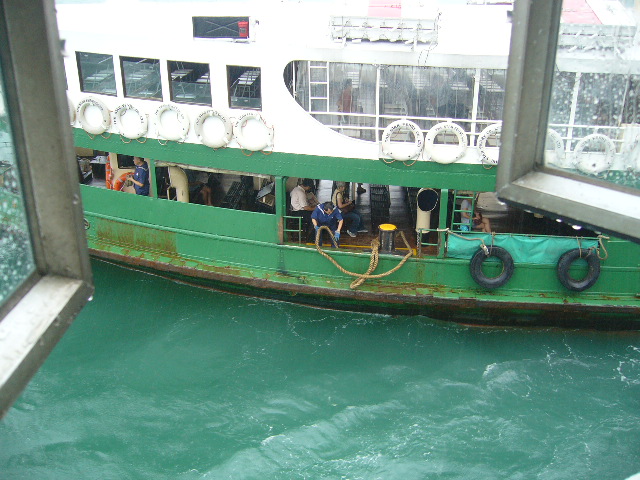This full-color square photograph, taken during the day, captures a detailed scene of an old ferry boat from a vantage point inside a building, through an open window. The boat features a rusted green lower hull and a white upper deck, with numerous white life preservers lining the sides. A crew member dressed in blue, sporting blue gloves, is holding a heavy rope, seemingly preparing to moor the boat to the dock. The lower deck has a yellow base where the rope is likely to be secured. On the far left, a man carries an orange inner tube, while two black tires hang as bumpers on the right side. Above, four square windows and a wider open door provide glimpses of ferry passengers and crew. The upper right windows reveal more individuals, suggesting a bustling atmosphere on board. The clear, greenish water below and the absence of the sky sharpen the focus on this quintessential ferry boat scene.